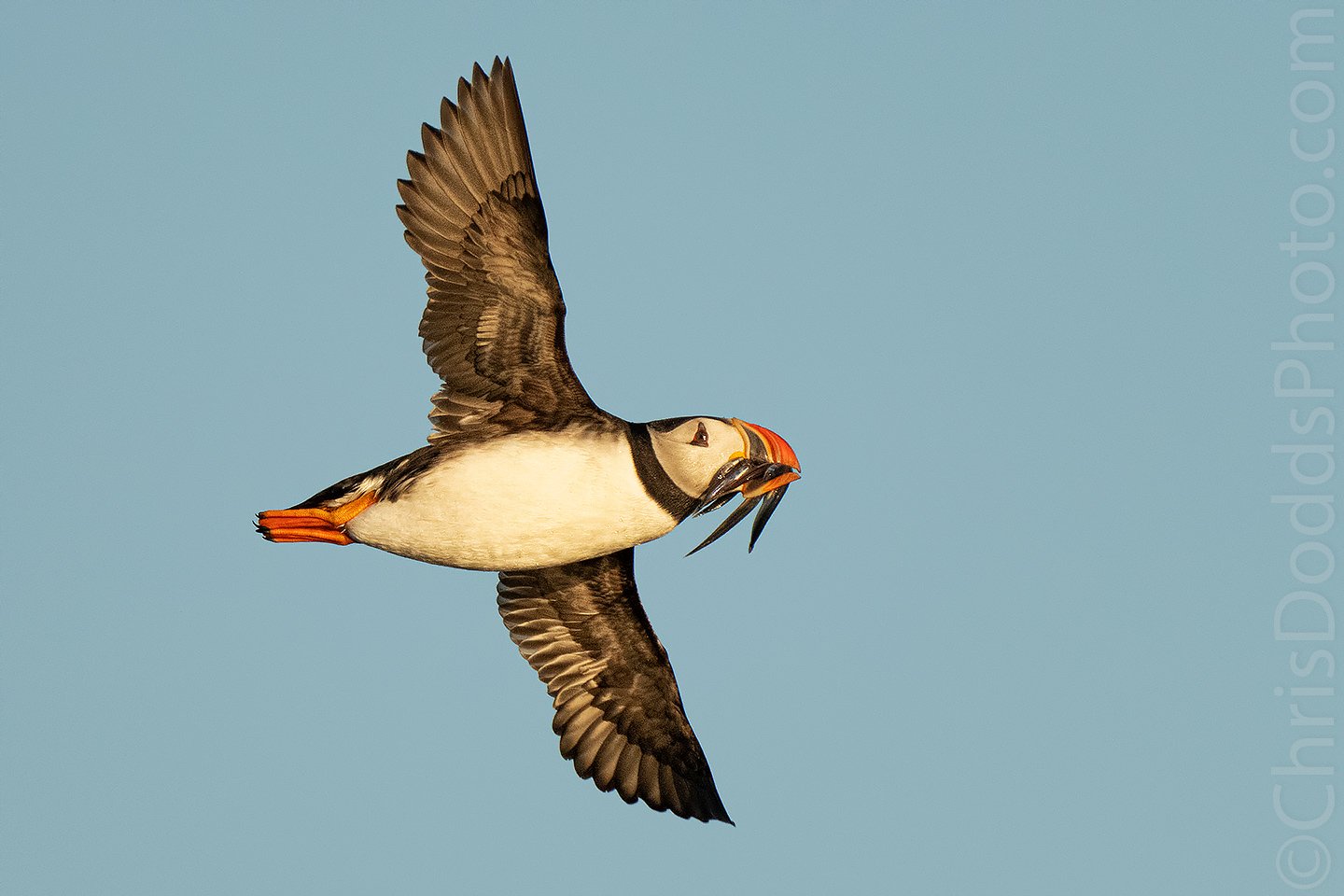This detailed photograph captures a penguin mid-flight against a bright blue sky. The bird, with its wide-spanned wings, showcases a stunning array of colors. The wings are predominantly dark but include lighter colored feathers, appearing grayish-black. The penguin’s round white belly and chest are prominent, with a distinctive black or brown line around its neck. Its small orange feet are spread out behind it, adding to the dynamic sense of movement. The bird's head is mostly white with a black eye and is adorned with a long, pointy beak that is an impressive mix of orange, yellow, and black. Observing closely, the penguin appears to be carrying something that looks like silver leaves or possibly small fish in its beak. The photograph includes a vertical watermark along the right side that reads "chrisdoddsphoto.com," confirming the photographer's credit.